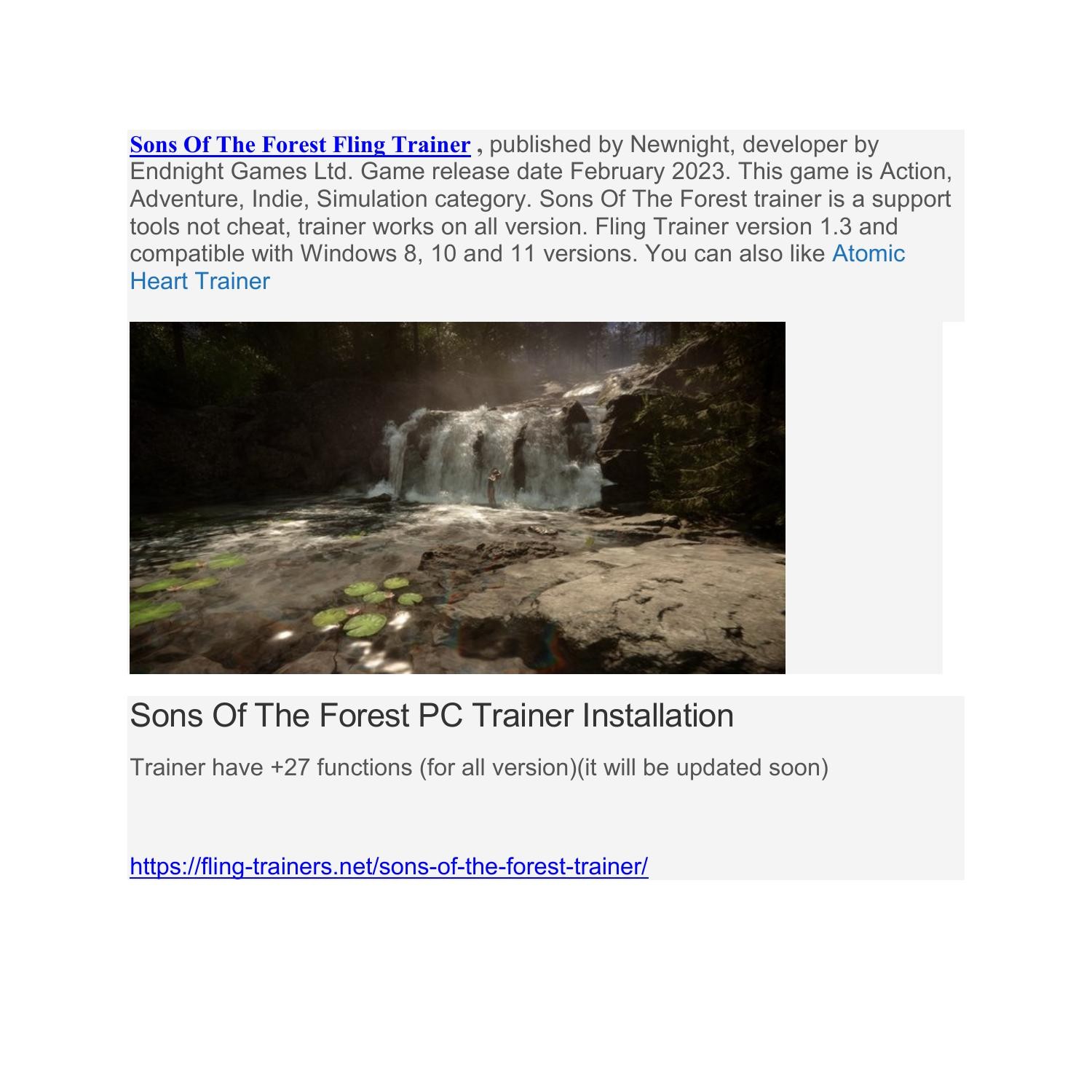**Caption:**

This image, seemingly sourced from a website, features a detailed overview against a gray background. At the top, a paragraph of text begins with a blue, underlined title, *Sons of the Forest Fling Trainer*. The subsequent text is black and reads: "Published by New Night, developed by In Night Games, LTD. Game release date February 2023. This game falls under the action, adventure, indie, and simulation categories. Sons of the Forest Trainer is a support tool, not a cheat. The trainer works on all versions. Fling Trainer version 1.3 is compatible with Windows 8, 10, and 11." The text then includes a recommendation: "You might also like Atomic Heart Trainer," where *Atomic Heart Trainer* appears in blue.

Below this text, the image shows a blurred graphic, predominantly black and white, depicting an outdoor setting with water and gray rocks. Green elements, possibly resembling lily pads, are situated at the bottom middle. Beneath the graphic, on a gray border, there is additional text: "Sons of the Forest PC Trainer installation. Trainer has over 27 functions for all versions. Updates will be provided soon." A clickable website link in blue is displayed under this information.